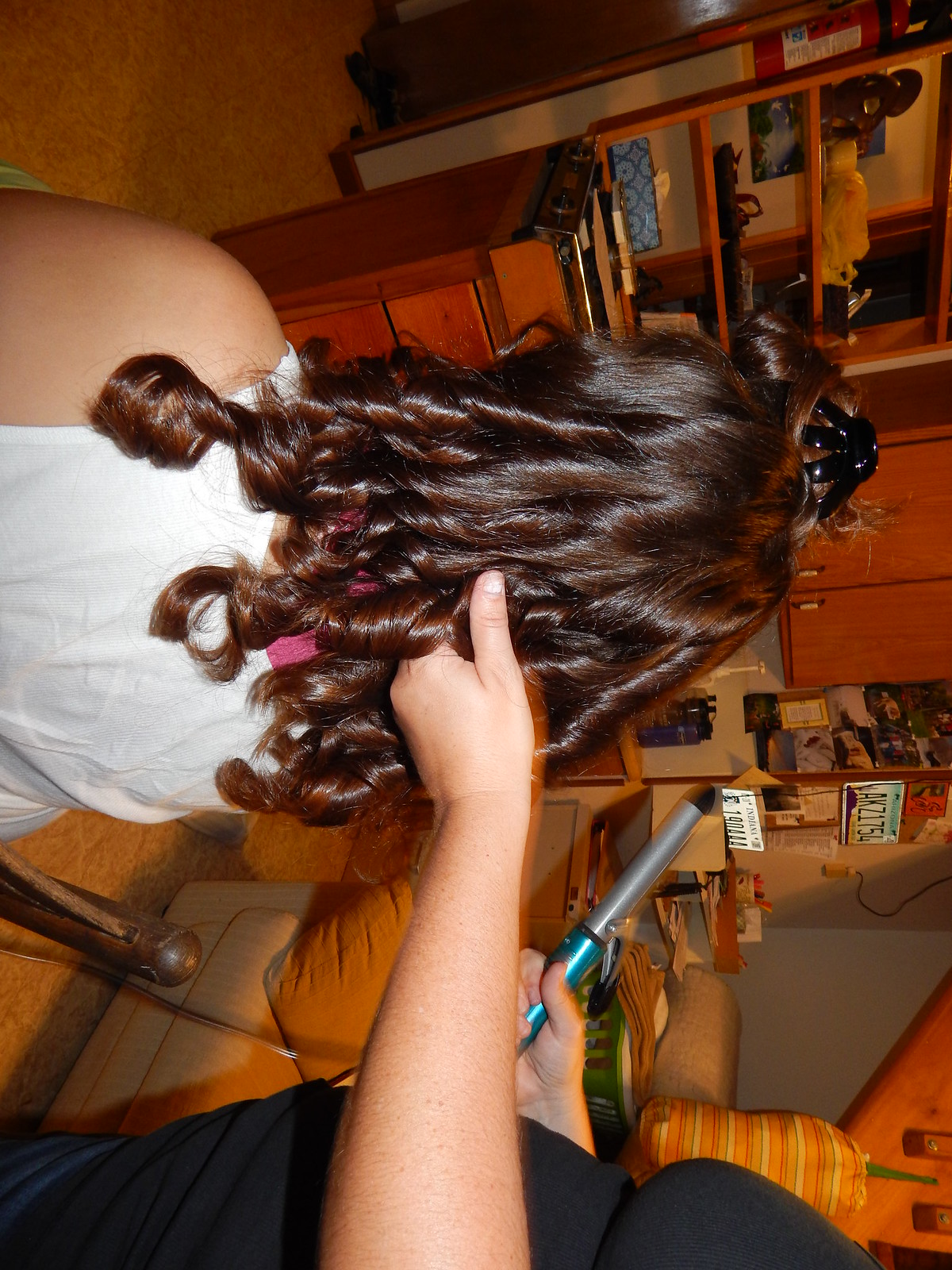The digital photograph, taken indoors with a vertical orientation, showcases a detailed scene of a living room office area featuring two Caucasian women. The focal point is a girl with dark brown hair, dressed in a white spaghetti strap tank top, getting her hair curled into ringlets using a curling iron. The curling iron has a silver barrel with a blue handle and is plugged in, held by another woman who is dressed in a black t-shirt and jeans. The girl sits straight-backed in a chair, leaning slightly forward, concentrating on the curling process being done from about midway down her scalp, making her hair hang in ringlets past her shoulders.

The living room has a beige, yellowish-tan carpet and various furnishings, including a couch with a yellowish pillow, a desk, cupboards, wooden counters with drawers, and bookshelves. There’s notable clutter on the small table stand and the walls are adorned with numerous knick-knacks and taped items, including an Arizona license plate with the number AKZ-1754. The carpet and furniture arrangement suggests a typical household setting, possibly indicating the girl is getting ready for an event, like a dance. The photograph's unique vertical perspective adds a quirky element, making the floor and furniture appear at the top of the image.